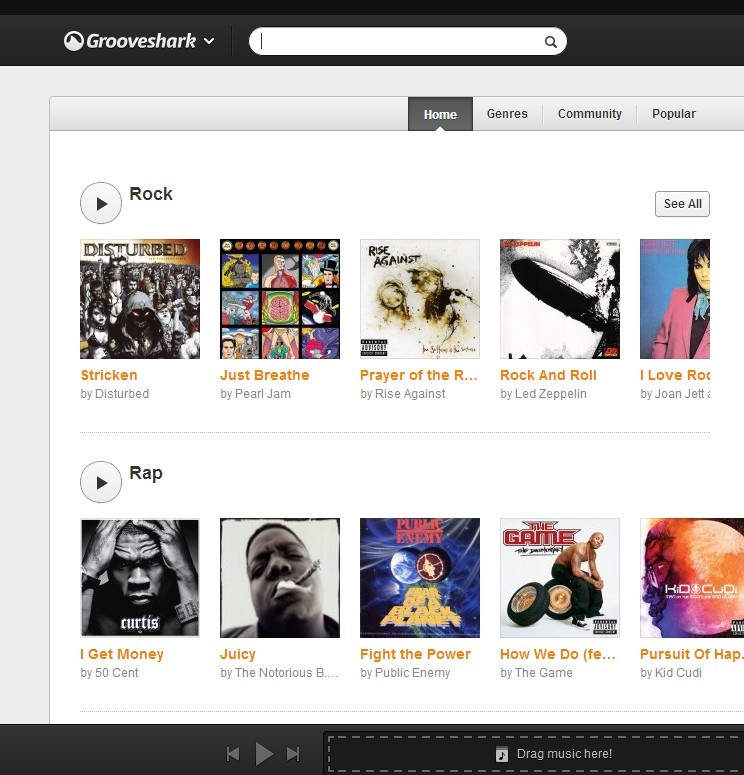The image depicts a screenshot of the Grooveshark music streaming platform. The upper left corner features the Grooveshark logo in white text against a black background, accompanied by a dropdown menu arrow. Dominating the top part of the interface is a large search bar with a magnifying glass icon.

In the top center, several navigation tabs are visible including Home, Genres, Community, and Popular, with the Home tab currently selected. Below these tabs, the screen showcases music albums categorized under the Rock genre. The first album on the left is "Districken" by Disturbed, featuring a cartoon-style drawing of a concert or rally. Next is "Just Breathe" by Pearl Jam, displaying six animated images. The third album, though its title is partially cut off, appears to be "Prayer of the Refugee" by Rise Against with a complex, hard-to-decipher cover filled with random dots. "Rock and Roll" by Led Zeppelin features an indistinct image of a person possibly holding a guitar. The last album in this row is "I Love Rock 'n Roll" by Joan Jett, showing Joan Jett in a pink blazer.

Another section below the Rock category is dedicated to Rap albums. This includes "I Get Money" by 50 Cent, with a cover of a man holding his forehead; "Juicy" by The Notorious B.I.G., partially cut off and showing him with a cigar; "Fight the Power" by Public Enemy; "How We Do" by The Game, featuring him sitting on tires; and "Pursuit of Happiness" by Kid Cudi, with his face emerging from a sun-like image.

At the bottom of the screen, there is a section labeled "Drag your music here," indicating users can add music to their library by dragging album covers into this area.